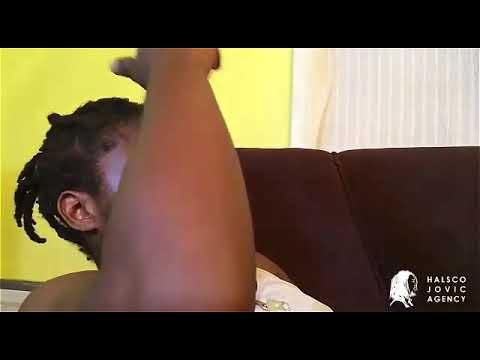A black man with short dreadlocks is reclining backward on the edge of a brown couch, his right arm raised and covering most of his face. His forearm extends upwards, nearly out of the frame, partially revealing the top of his head and a small portion of his ear catching some light. He is wearing a white shirt, possibly featuring an embossed design or a necklace that resembles a peace sign. Behind him, the wall is painted yellow, contrasting with a white curtain adorned with vertical lines on the right. In the bottom right corner of the image, white text reads "Alsko Jovik Agency" alongside a white decal depicting a person adorned with a headscarf and a mask over their shoulders.